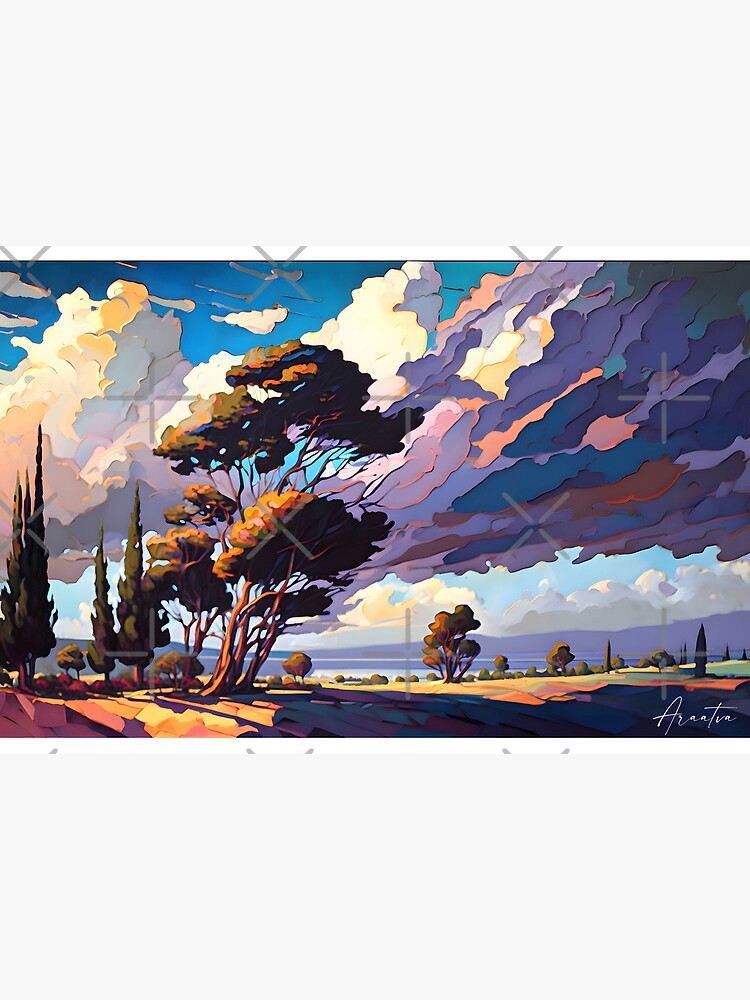This image is a vibrant digital watercolor landscape depicting various elements of nature. In the foreground, there is a mix of flat sandy terrain with patches of bright and dark colors, creating a distinctive blocky effect. Tall, slender trees, including pine and acacia-like varieties, are scattered across the scene, with some appearing to sway as if blown by the wind. In the background, a large tree with dense branches adds depth, and a faint slope rises to the right.

Above, the sky shifts from light to dark blue, filled with dynamic clouds ranging in hues from white and yellow to deep purples and blues, illustrating possible sun patterns or weather changes. The clouds show intricate details, with lighter, fluffy formations on one side transitioning into darker, more ominous shades on the other. A body of water can be glimpsed at the horizon, adding a serene blue to the mix of colors.

The artwork prominently features the artist's signature in the bottom right corner, starting with an “A,” and is accompanied by transparent watermark X's. Despite its detailed and possibly desert-like characteristics, the landscape combines elements of both sandy and lush environments, framed by a vivid representation of the sky and cloud dynamics.